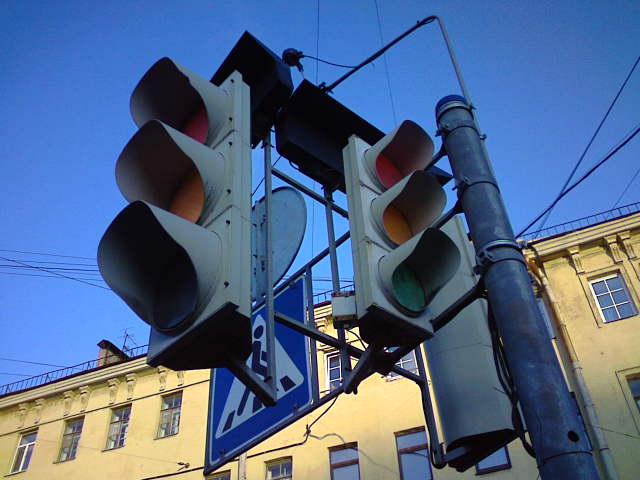This color photograph, taken from a low angle looking upward, captures a pair of traffic lights mounted on a dark gray pole. Both traffic lights are encased in an off-white metal and comprise the standard red light at the top, orange in the middle, and green at the bottom, though none of the lights are currently illuminated. One of the traffic lights is angled to the upper left, while the other is oriented to the upper right, with an additional light facing the opposite direction. Adjacent to the traffic lights is a blue pedestrian crossing sign featuring a white triangle and a black stick figure crossing a street.

In the background stands a yellow building with several small windows arranged in a row, adorned with decorative buttresses beneath its edge. Some windows reflect the clear blue sky above, which displays a rich, deep shade of blue with no clouds. The perspective also hints at architectural details like small iron gates, adding to the urban scene's richness and intricacy.